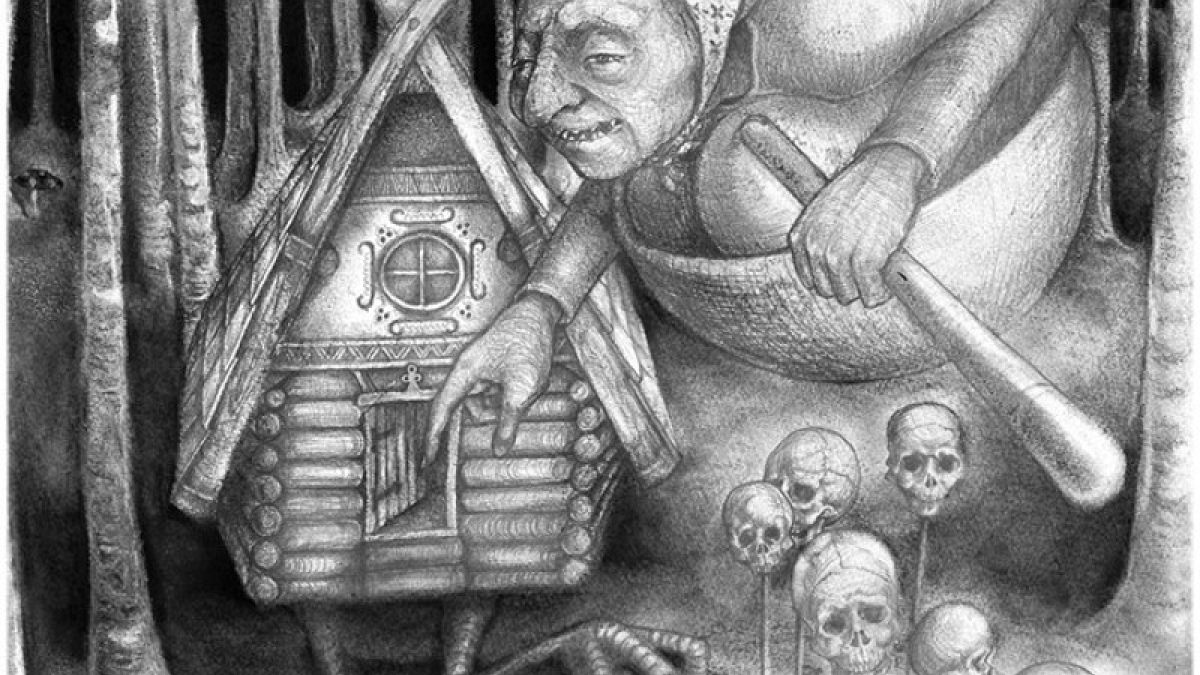This eerie black and white digital illustration depicts a sinister scene set in a dark forest. Central to the image is a large, grotesque figure that combines features of a troll and a gnome. It wears a hat tied under its chin and crouches awkwardly inside a spherical chair, grasping a wooden stirring stick, resembling a baseball bat, in its left hand. With its other hand, it ominously opens the door of a small, quaint log cabin that is precariously perched on bird-like claws. The creature's exaggerated features, including a large nose and menacing presence, signify it wouldn't fit inside the tiny house. Around the cabin, eerie details elevate the unsettling atmosphere: the right side of the cabin is adorned with human skulls mounted on sticks, while the left side is cluttered with gnarled tree branches and trunks. The entire scene is imbued with a dark, creepy vibe, suggesting a world filled with malevolent fantasy elements.